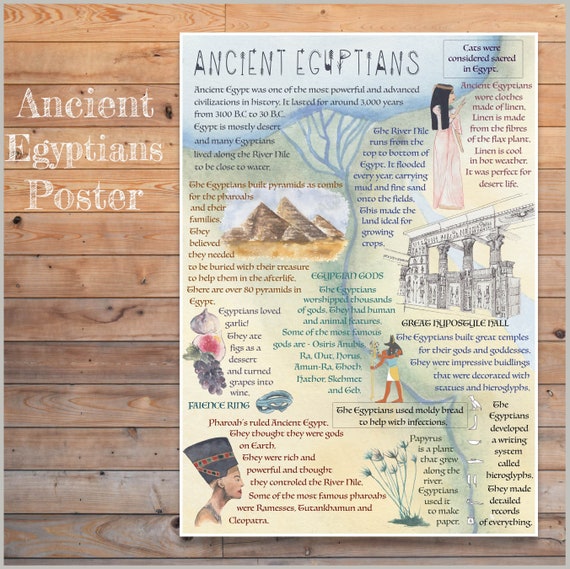This photograph captures a detailed educational poster titled "Ancient Egyptians," prominently displayed on an unfinished wooden surface composed of rows of planks. The primary background of the poster features a map of the Nile River, symbolizing its crucial role in ancient Egyptian civilization. At the top of the poster, bold white text reads "Ancient Egyptians." Below, a comprehensive passage begins with, "Ancient Egypt was one of the most powerful and advanced civilizations in history," providing a narrative about the nation's rich heritage.

Interstitial illustrations accompany the text, depicting significant figures and deities from ancient Egypt. These include an image of Anubis, the jackal-headed god associated with mummification and the afterlife, alongside a representation of a goddess whose identity is not explicitly clear. Among these illustrations is also a portrait of a pharaoh, epitomizing the rulers of this historic era.

In addition to these figures, the poster includes drawings of various food items integral to ancient Egyptian culture, such as garlic, figs, and grapes. These elements contribute to a vivid portrayal of daily life in ancient Egypt.

The photograph seems to be captured in natural lighting, though it remains ambiguous whether the setting is indoors or outdoors, or whether the image itself is a digital rendering. The attention to detail in both the poster and the wooden background offers an informative and visually engaging glimpse into the world of the ancient Egyptians.